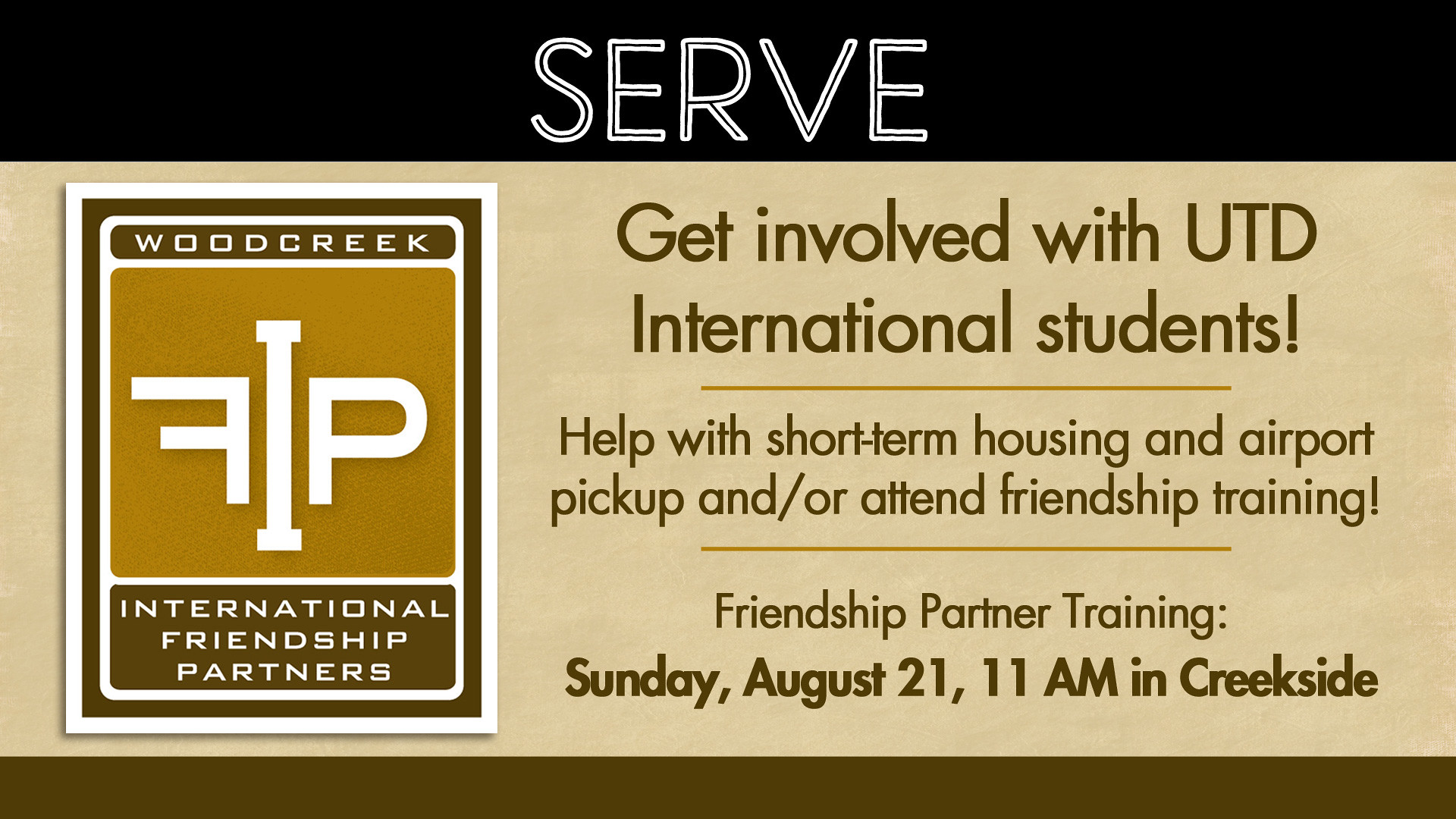The informational poster is a horizontally-oriented advertisement featuring various text sections and imagery. Dominating the top of the poster is a long black bar, within which the word "serve" is prominently displayed in white capital letters, each letter bisected by a thin black line to emphasize the text's clarity. Below this, against a light tan background, the poster invites viewers to "get involved with UTD international students" in light green lettering. The subsequent content, in dark brown font, suggests ways to participate, such as providing short-term housing, assisting with airport pickup, and/or attending friendship partner training. Specific event details are also included: "Sunday, August 21, 11 a.m. in Creekside."

To the left side of the poster, an orange logo features the letters F, I, and P, with the F appearing to be backwards and the I and P in white. Above the logo, the words "Wood Creek" appear in white, while below it reads "International Friendship Partners." The bottom of the image is marked by a long vertical dark brown bar with the word "serve" repeated, using the same stylistic black line through each letter as featured at the top of the poster.